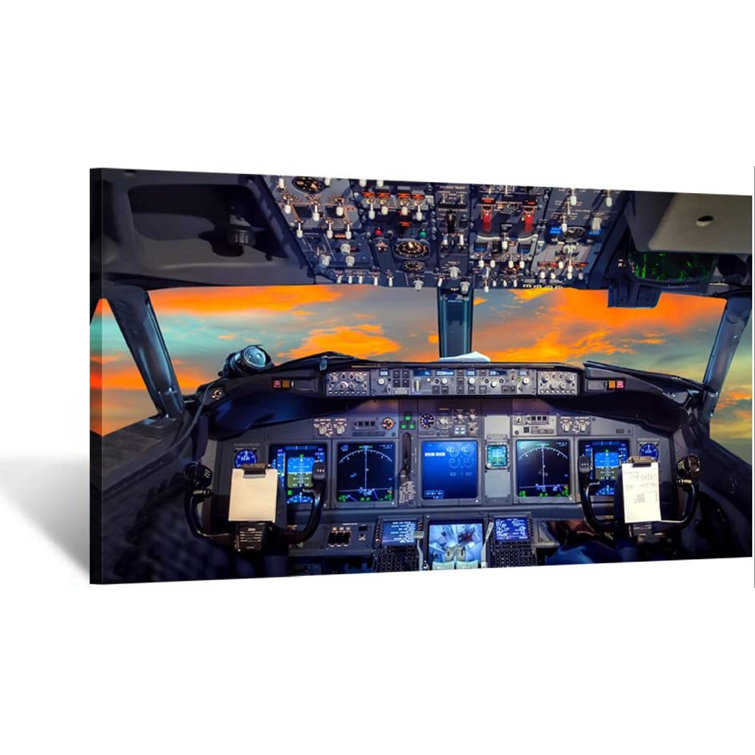The photograph captures an intricate and realistic airplane cockpit, potentially in a simulator or an actual aircraft. The cockpit is detailed with numerous buttons, knobs, and toggle switches, predominantly at the top section of the control panel, which features white and red switches. Spread across the cockpit are several display screens, most of which have a blue theme with detailed white lines, and are framed by a surrounding gray area. The cockpit interior appears dark with a grayish-blue hue. Visible through the cockpit windows are vibrant sky scenes with blue skies and striking orange and yellow clouds, suggesting it is daytime. Central to the cockpit are the black steering handles for the pilots, and two white clipboards with papers can be seen positioned in front of the pilot seats. The image is sharp and brightly illuminated by natural light, lending a clear view of both the cockpit details and the exterior scenery. Notably, no pilots or other individuals are present in the image.